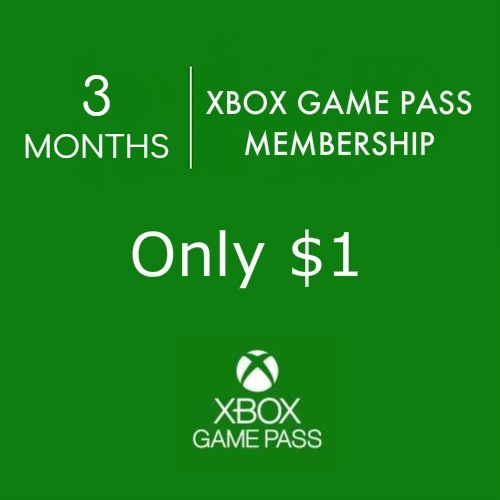The image features a rectangular design with a dark green background and white text predominantly displayed on the left side. At the top, large, bold, capitalized letters read "3". Directly below that, still in capital letters but in a smaller size, it says "MONTHS". This text appears in a rounded, Century Gothic-like font.

A white vertical line acts as a divider, separating this section from the content on the right side. To the right of the line, the text "XBOX GAME PASS MEMBERSHIP" is prominently displayed in bold, capital letters, matching the white coloration.

Below this, in larger sans-serif font reminiscent of Calibri, the word "ONLY" appears, followed by a dollar symbol and the numeral "1", indicating a promotional price of $1. The "1" features a distinctive typographic style, with a short diagonal tail at the top and a base line at the bottom.

Beneath this pricing information is the iconic Xbox logo: a white circle with a stylized "X" whose legs wrap around the sphere to give a 3D effect. Under the logo, the word "XBOX" is written, with the middle line of the "B" extending slightly to the right, overlapping its vertical line. Following this, it says "GAME PASS" in capitalized, white letters, maintaining the overall bold, clean aesthetic.

The detailed fonts and strategic layout emphasize the limited-time offer, creating a visually striking advertisement for the Xbox Game Pass membership.